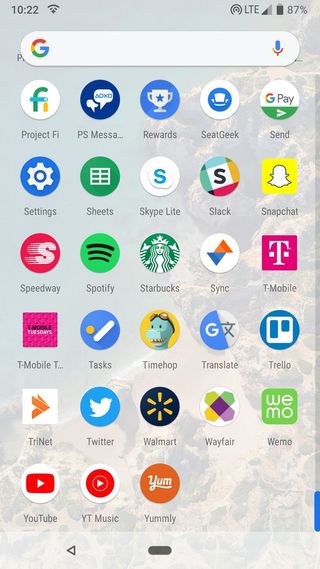The image displays a screenshot of a smartphone screen, encapsulated within the typical dimensions of a modern phone. In the upper left corner, the digital clock reads "10:22," next to a cell signal indicator and the "LTE" label in the upper right, showing about two to three bars of signal strength. Further to the right, the battery level is at 87%.

At the top of the screen, there's a Google search bar, complete with the iconic colorful "G" on the left and a microphone icon on the right. Below this search bar, numerous app icons are arranged in a grid. These include Project FI, PS Message, Reward, Seek, Geek, Send, GPay, Settings, Sheets, Skype Lite, Slack, and Snapchat.

Scrolling further down, additional app icons line the screen: Speedway, Spotify, Starbucks, Sync, T-Mobile (with even more entries for T-Mobile just beneath), Tasks, TimeHop, Translate, Trello, Trinet, Twitter, Walmart, Wayfair, WeMo. 

The bottom row features three prominent apps: YouTube, YT Music, and Yummly. At the very bottom of the screen, the navigation bar is visible, containing the standard left-facing arrow and a central oval icon, all set against a translucent stripe.

The wallpaper in the background is subtly elegant, depicting what seems to be a cliff or an underwater rocky shoal. This faint yet beautiful background does not distract from or obscure the array of app icons laid over it.